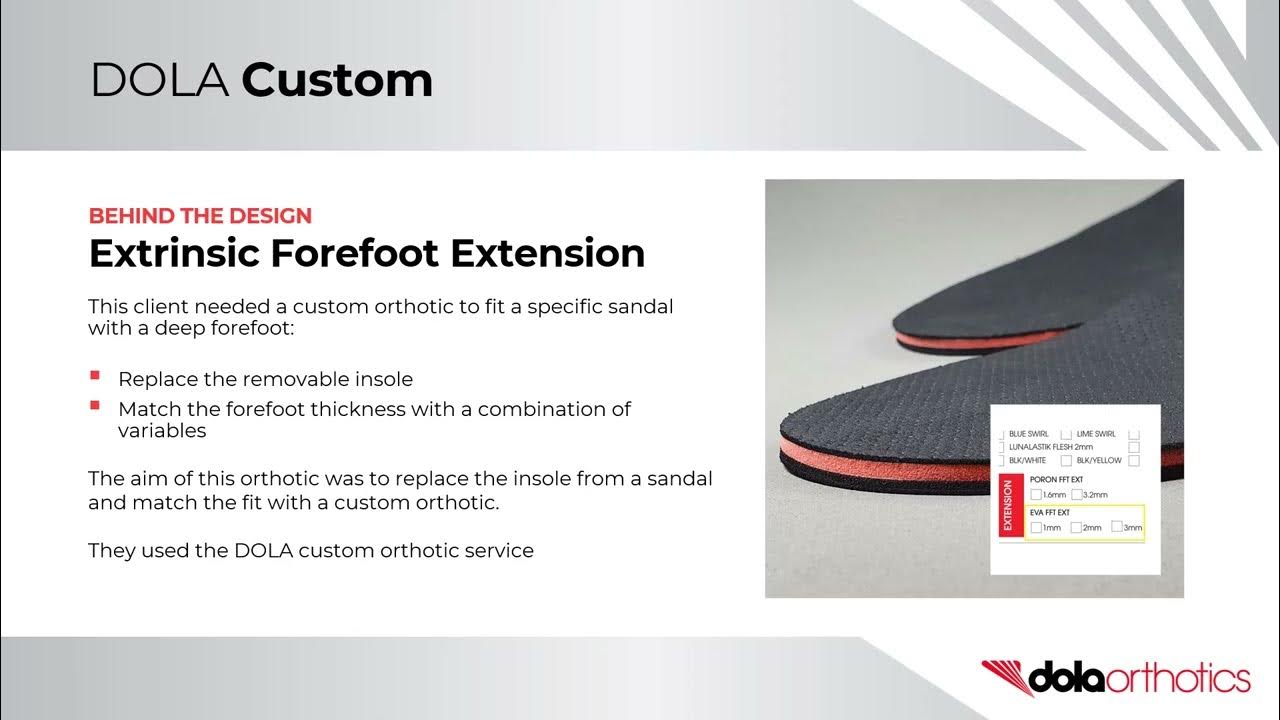The image is an informative poster showcasing custom orthotic insoles from DOLA Orthotics. At the top, a gray banner with diagonal gray stripes on the right side displays the text "DOLA CUSTOM" in thin capital letters and bold black font, respectively. Centrally featured in a large white rectangle, the phrase "Behind the Design" is presented in red lettering, followed by the phrase "Extrinsic Forefoot Extension" in bold black letters. The information explains that the client needed a custom orthotic to fit a special sandal with a deep forefoot. Below this are two red bullet points: the first advises to replace the removable insole, and the second to match the forefoot thickness using a combination of variables.

To the right, a square image showcases the orthotics, characterized by a black top layer, a red foam layer in the center, and a black bottom layer. A white box within this section includes black text mentioning specific details about the orthotic's design, although the text is too small to make out all the details clearly. At the very bottom of the poster, the brand name "DOLA Orthotics" appears in black and red lettering, accompanied by their reddish logo.